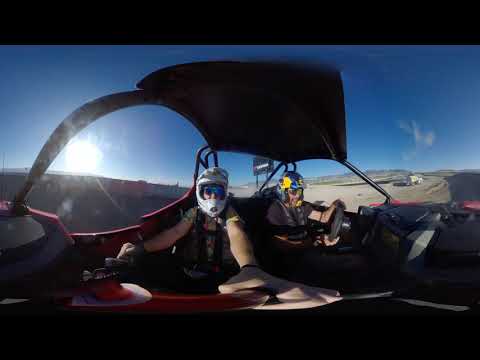The image captures the interior of a sand buggy or similar adventure sports vehicle from a vertical rectangular perspective. Framed with horizontal black stripes at the top and bottom, the scene depicts two individuals seated and fully engaged in operating the vehicle. Each person is equipped with a helmet and goggles, their faces obscured, and they are strapped in with black harnesses for safety. The person on the left wears a white helmet, blue goggles, and possibly a yellow-green shirt, while the individual on the right dons a yellow and blue helmet, black glasses, a black shirt, and jeans. Both appear to be working controls with arms outstretched.

The interior of the vehicle showcases a black and red dashboard and a partially visible steering wheel, suggesting both occupants are involved in the vehicle's operation. The roof is black, and the interior appears red. A clear plastic cover envelopes the occupants, offering an unobstructed view of the outside environment. Below this cover, the ground slopes away beneath the horizon, with a gray, curved surface merging into a body of blue water dotted with white clouds to the right.

In the backdrop, a bridge, likely gray and sunlit to the point of near-opacity, spans from the left to right, carrying vehicles. The bright, white sun hovers on the lower left, casting daylight across the scene, which is further accentuated by the clear blue sky overhead. A black sign with indistinct white text, possibly hinting at a brand like Verizon, is also visible in the background.